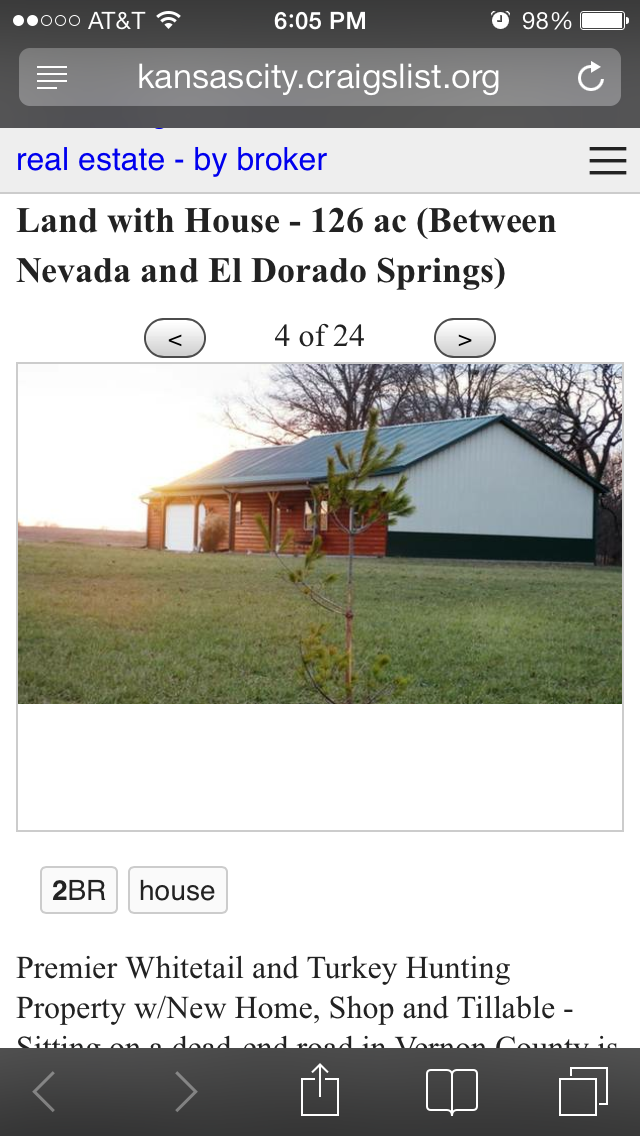This is a detailed screenshot from a phone displaying a real estate listing on the Kansas City Craigslist site, with the URL "kansascity.craigslist.org" visible at the top. The service provider is AT&T, Wi-Fi is enabled, the time is 6:05 p.m., and the battery is at 98%. The listing advertises "Land with House, 126 Acres" located between Nevada and El Dorado Springs, specifically in Vernon County, on a dead-end road. The property includes a new home, a shop, and tillable land, and is ideal for whitetail and turkey hunting.

The screenshot captures the fourth image out of 24 available pictures in the listing. This image shows a house with a white side and green or black roof, and a log front. The yard features grass, a small pine tree in the foreground, and larger trees in the background. The interface of the phone reveals a blue link indicating the real estate section, and options for going forward and backward through the images. The bottom part of the screen includes standard phone navigation options and buttons for sharing or bookmarking the listing. The page's background is the usual Craigslist white with black text, and the real estate link highlighted in blue.